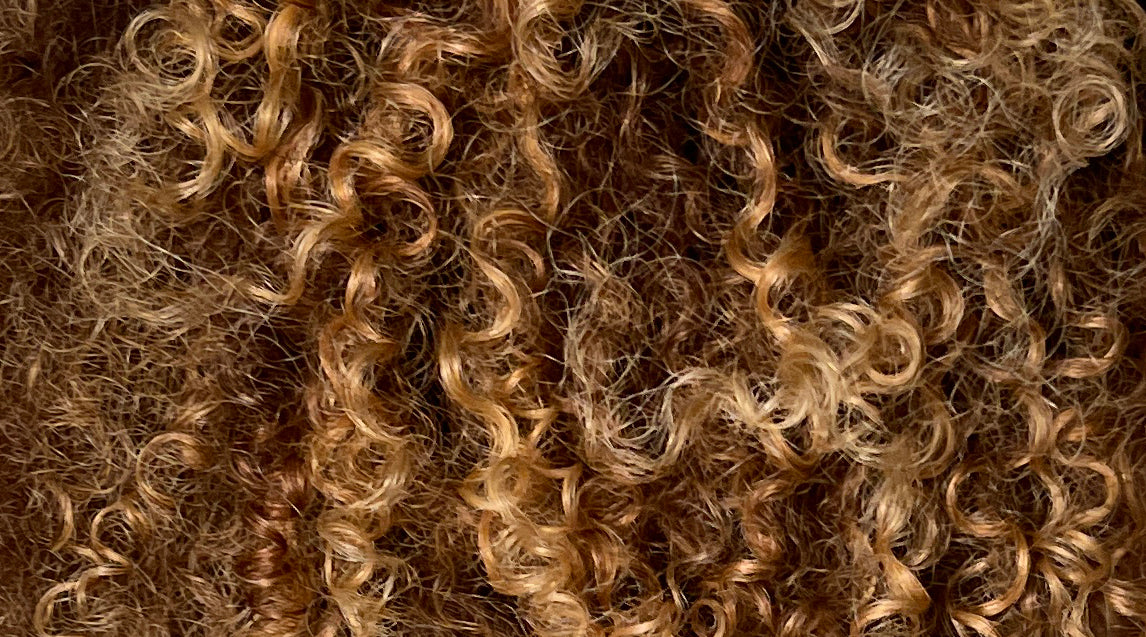The image depicts a close-up view of long, curly hair, captured in a landscape perspective that's approximately 1.5 times wider than it is tall. The hair appears scattered yet organized, primarily flowing from north to south. It's predominantly light brown in color, though it exhibits variations, with strands of light blonde and reddish-brown tones present. At the center of the image, the hair is densely packed with defined curls, giving it a structured appearance. Moving towards the edges, especially on the left side, the curls become less pronounced and the hair appears frizzier and somewhat straight, but still messy. Light also interacts with the hair, emphasizing its texture and color variations. Despite the messy appearance, there's a notable contrast between the densely curled sections in the center and the straighter, more unruly strands towards the outer areas.